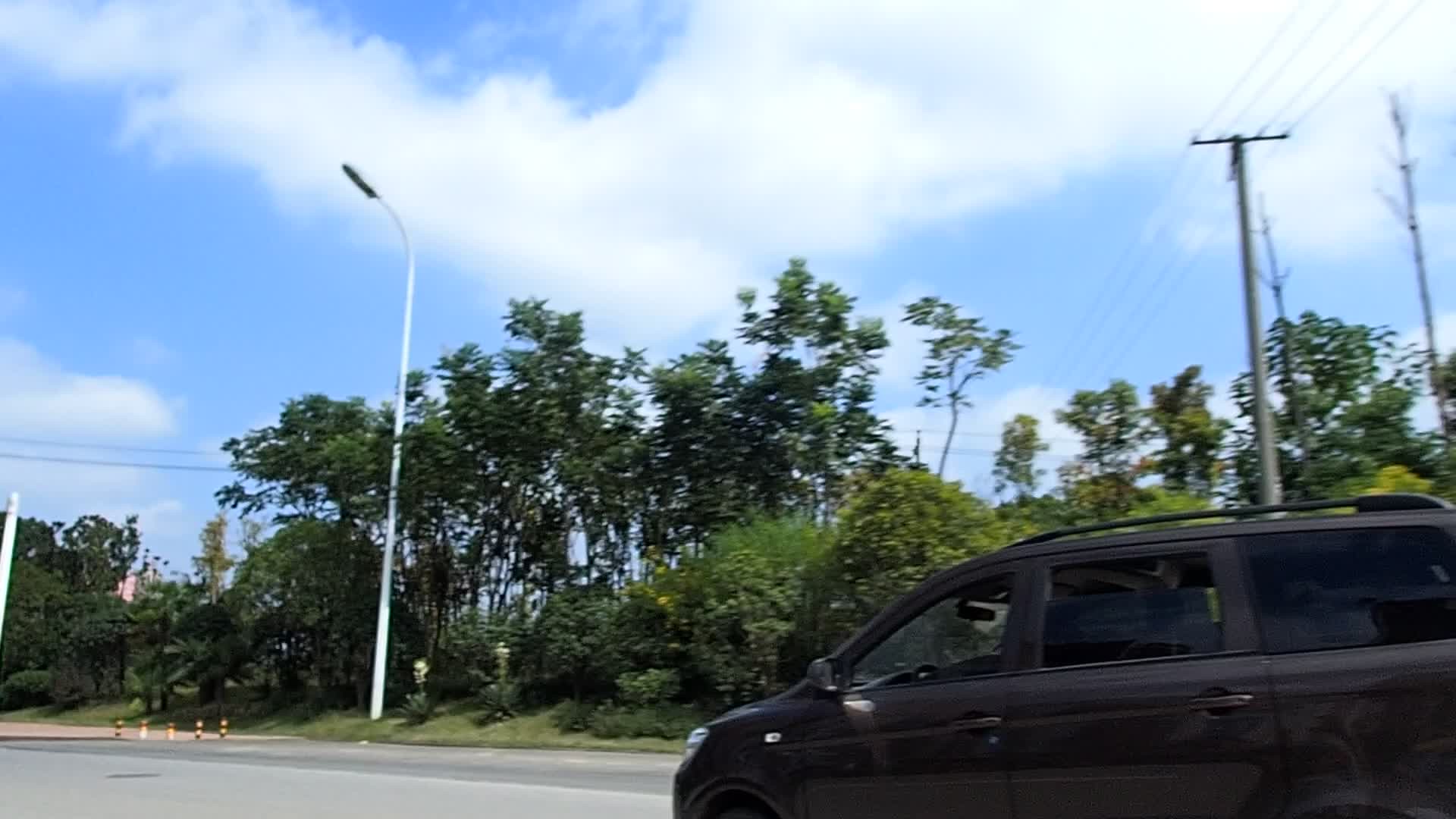This is a detailed photograph taken from a moving vehicle's passenger side window, capturing a dynamic scene on a wide road. The focal point is a black minivan with tinted windows and the driver's window rolled down, traveling parallel to the photographer's vehicle. The van's specific make is unclear, but it suggests a Chrysler or Dodge model. In the bright, sunny daylight, a vividly blue sky dotted with fluffy white clouds covers about two-thirds of the upper frame, casting a serene backdrop over the scene. Surrounding the road are lush green trees, shrubs, and power lines running alongside, supported by both a utility pole on the right and a white street lamp on the left. Additional roadside elements like a protective barrier and a sidewalk are faintly visible, emphasizing the well-populated and maintained green area through which the vehicles are traveling.